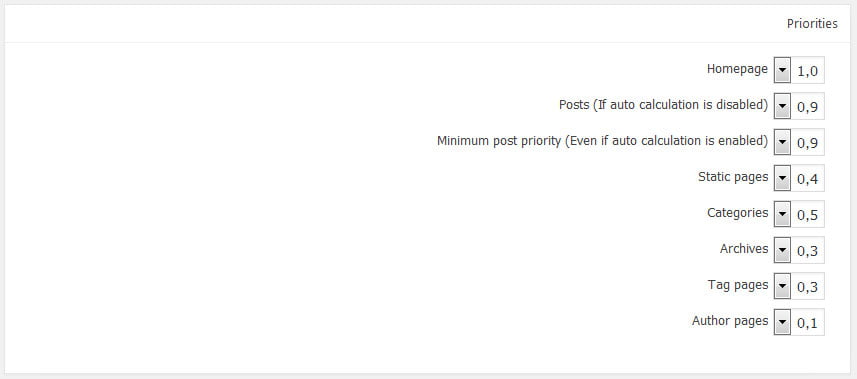This image displays a page containing a list of text items detailing various priorities and settings for a website's content organization. On the right side of the page, the text outlines the following:

- "Priorities: Posts" – indicating the ranking or importance assigned to posts.
- "If auto-calculation is disabled" – specifying conditions for manual adjustments.
- "Minimum post priority" – defining the lowest priority level for posts.
- "Even if auto-calculation is enabled" – suggesting that certain settings apply regardless of automatic calculation.
- "Static pages" – referring to non-dynamic pages on the website.
- "Categories" – likely indicating how content is categorized.
- "Archives" – referring to the storage or organization of past content.
- "Tag pages" – pages that organize content based on tags or keywords.

The text collectively provides insight into how different types of content are prioritized and managed within the system.